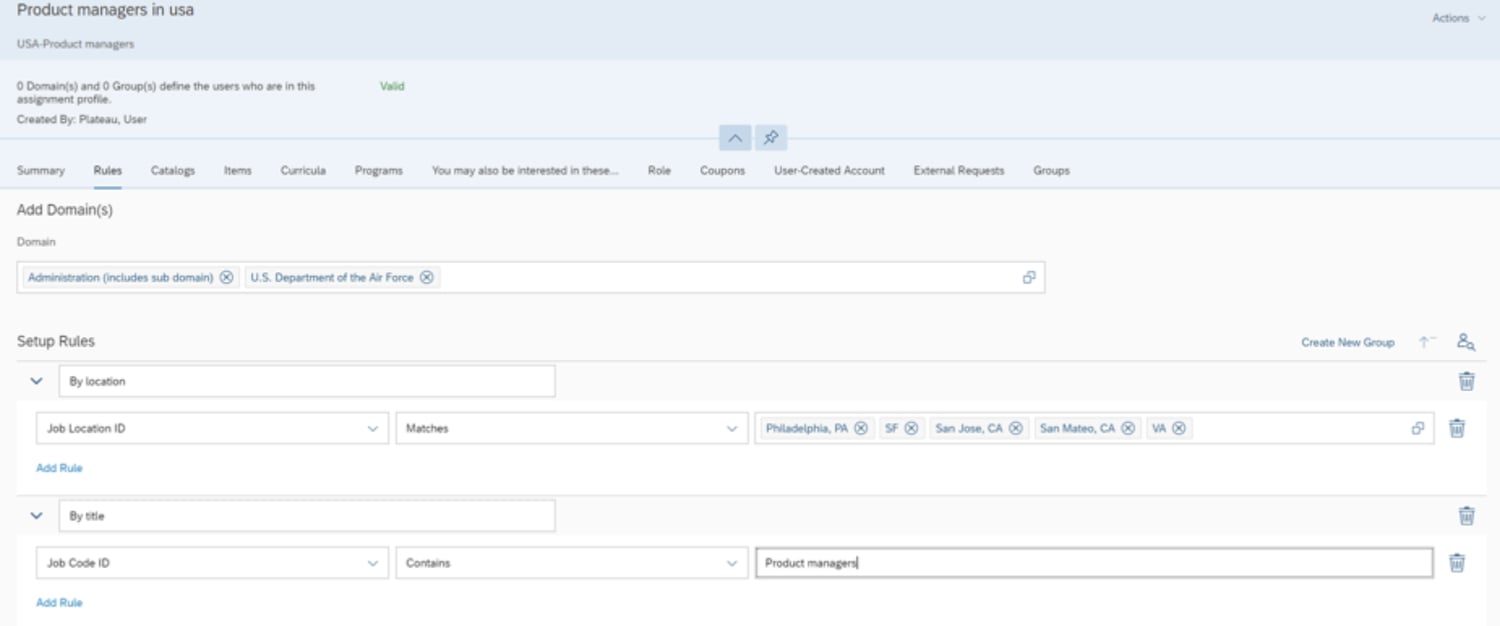This screenshot appears to be from a software or website interface, likely related to user or role management within an organization. The top third of the screen features a pale blue background with the title "Product Managers in USA" in black text. Below this header, it confirms the context with the text "USA – Product Managers."

Further down, black text indicates that there are currently "Zero Domains and Zero Groups defined" for the users included in this assignment profile, which was created by a user. A green text status alert indicates that this assignment profile is valid.

Underneath this section, there are several tabs for navigation: Summary, Rules, Catalogs, Items, Curricula, and Programs. There are also additional navigation options provided, including: Roll, Coupons, User Created Accounts, External Requests, and Groups.

The background then transitions to a pale gray, where it reads "Add Domains" under the "Domain Administration" heading, specifically mentioning "US Department of the Air Force."

Further down, there is a "Setup Rules" section. Here, rules can be configured:
- By Location: Job Location ID matches Philadelphia, PA; San Francisco, CA; San Jose, CA; San Mateo, CA; or Virginia.
- There is an option to add more location-based rules.
- By Title: Job Code ID contains "Product Managers."
- Additional title-based rules can also be added.

The interface seems to be geared towards setting up and managing user profiles and access based on specific rules and domains, likely for an organizational or administrative purpose.